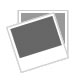This image is a highly magnified photograph featuring two metal objects, set against a black background. On the right, there's an extreme close-up of a coin, likely a quarter, with only the left-hand rim and the letters "LI" visible. The magnification reveals minute scratches and wear, indicating extensive use over time. On the left, there is a polished, gold-colored clasp attached to what appears to be a piece of jewelry or machinery. This clasp includes silver or white-gold wires wrapping around a central point, with a curved edge that descends to the left. The extreme zoom of the photo makes some details blurry and pixelated, emphasizing the intricate textures and reflective surfaces of the objects. The juxtaposition of the coin and the clasp suggests that the quarter may be included for scale, highlighting the small size and fine craftsmanship of the adjacent item.